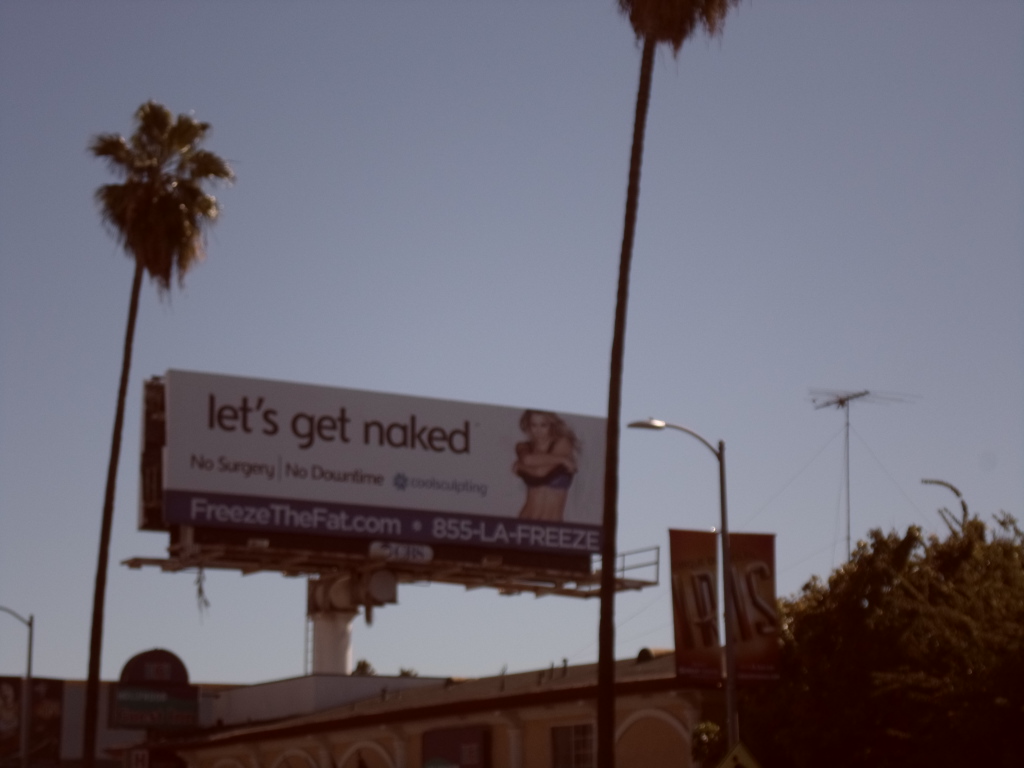The photograph captures a slightly wider-than-tall billboard on the side of the road, framed by two tall palm trees extending higher than the billboard itself. The scene offers an urban, Southern California vibe with a clear blue sky, a light post, an antenna, and power lines in the distance. The billboard, predominantly white with a blue band at the bottom, features bold black text reading "Let's Get Naked" followed by "No surgery. No downtime." On the right side of the billboard, a Caucasian woman is depicted in the process of removing her top, revealing a bare midriff and wearing a bra with her arms across her chest. The blue band at the bottom contains the website "freezethefat.com" and the phone number "855-LA-FREEZE". The overall photograph is slightly out of focus, but the main elements of the billboard remain discernible.